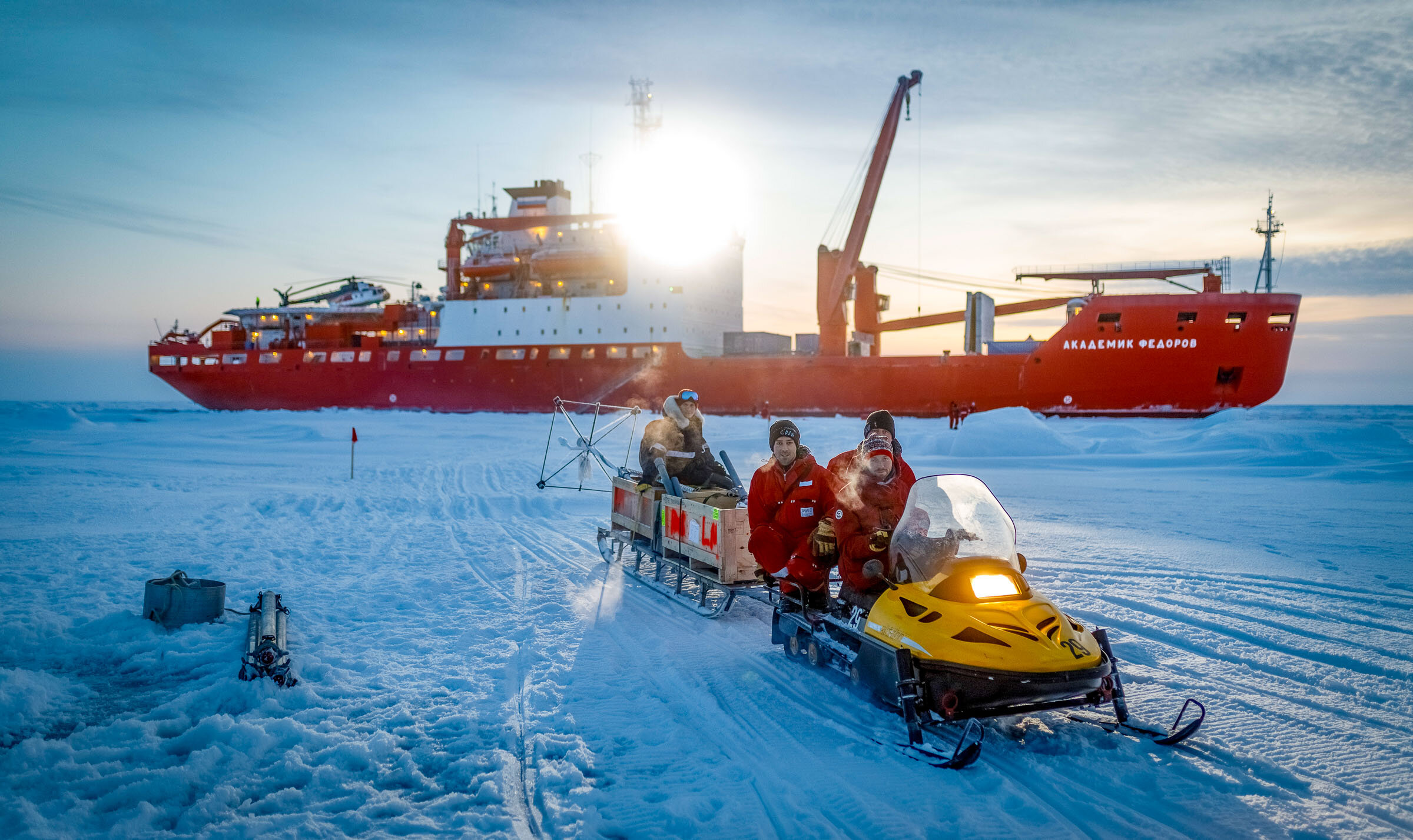In this detailed and evocative image captured in what appears to be the Arctic or far northern hemisphere, a vast expanse of snow and ice stretches to the horizon, meeting a desolate coastline. Dominating the background is a massive red ship, possibly a cargo or research vessel, adorned with Cyrillic script and equipped with a helicopter and cranes, suggesting it's stationed for significant operations. The vessel spans almost the entire width of the photo, with the sun casting a bright glare over its top edge, highlighting the stark, cold environment. In the foreground, we see a snowmobile designed for heavy snow conditions, bearing a headlight and towing multiple sleds laden with large boxes and equipment. Four people, all dressed in red uniforms with beanie caps, are riding the snowmobile and the sleds; their visible breath attests to the frigid temperatures. To the left, additional machinery is subtly visible amid the snow. The collective attire and equipment underscore the challenging, icy conditions of this remote and rugged landscape.